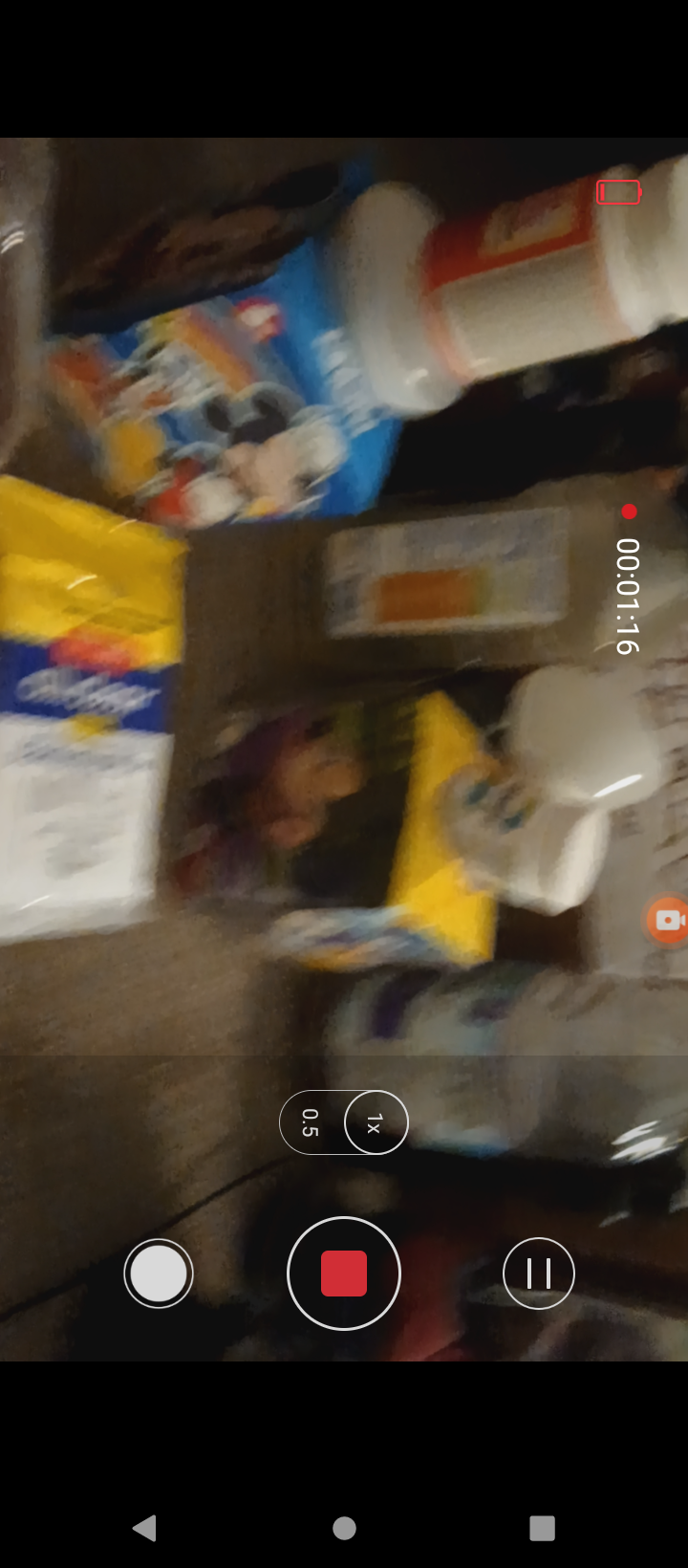This image appears to be a blurred and grainy screen grab from a cell phone, showing a side view of objects on a wooden table. The cell phone's recording interface is visible, with three circles at the bottom—one containing a red square indicating the record function, another with a white filled-in circle, and a third with two straight lines. To the right center of the screen, there’s a red dot and a timer displaying "00:01:16," suggesting the recording has been ongoing for a minute and 16 seconds. The background shows a cluttered table or counter, with several boxes and containers. Among these items, one box features a Mickey Mouse character and is blue in color, possibly a tissue box or food item. Another container, possibly a vitamin or pill jar, sits atop this Mickey Mouse box, surrounded by additional bottles. The table appears brown and shiny, contributing to the reflective nature of the surface.